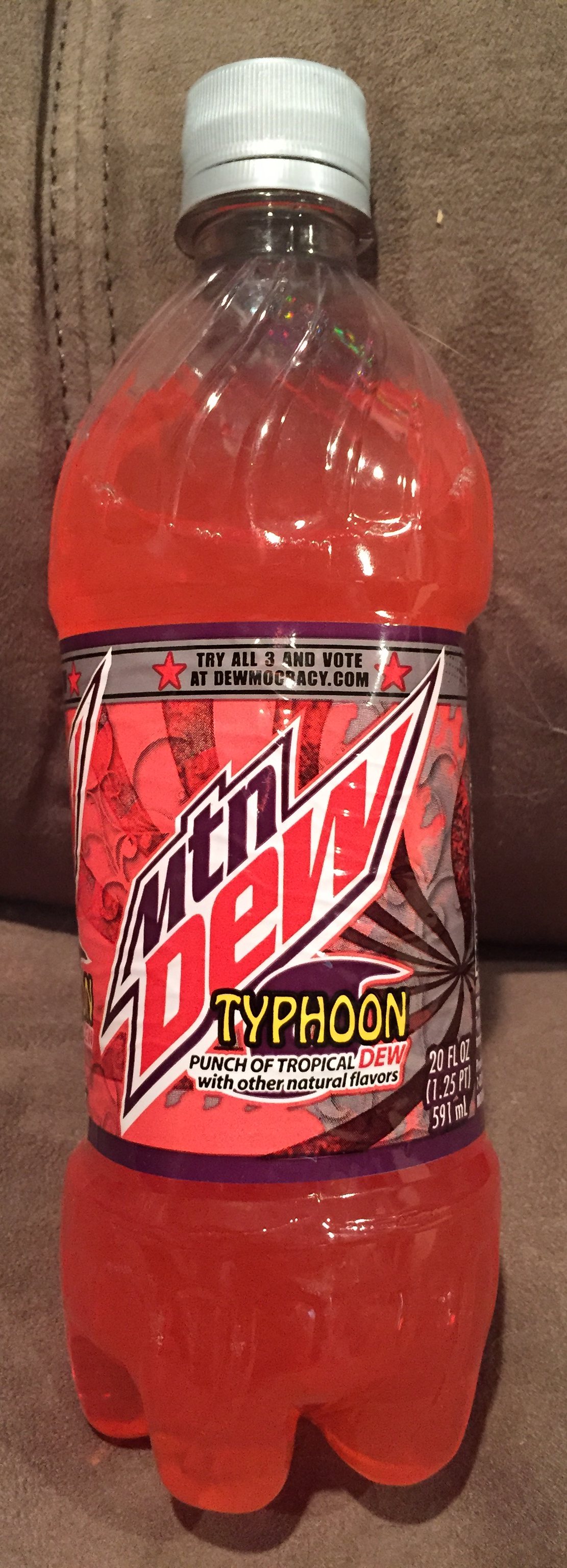The indoor image captures a stone granite countertop or table as its primary setting. Dominating the foreground is an unopened 20-ounce bottle of Mountain Dew Typhoon, a bright pink beverage. The bottle features a grey and pink label, with "Typhoon" prominently displayed in yellow letters. The cap is also grey, mirroring the label's color scheme. Leaning slightly against what appears to be a leather bag or briefcase in the background, the bottle's liquid tilts accordingly, giving it an off-kilter appearance. The leather item adds a subtle textural contrast to the otherwise crisp and vibrant focus on the Mountain Dew Typhoon bottle.